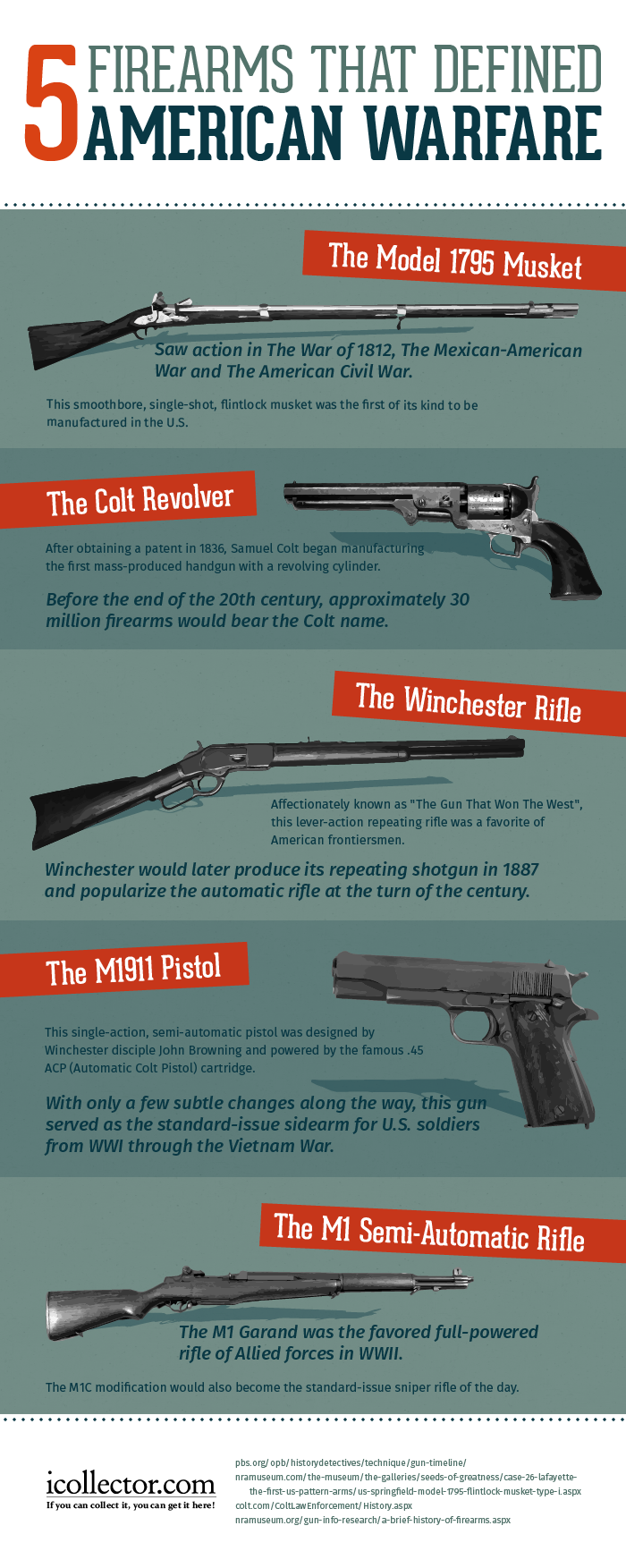This poster, shaped as a slender vertical rectangle, prominently features the title "FIVE FIREARMS THAT DEFINED AMERICAN WARFARE" in various colors: the numeral "5" in orange, "Firearms that Defined" in dark green, and "American Warfare" in a darker greenish-blue on a white background. Beneath the title, the poster is divided into five horizontally-oriented panels, each showcasing a different firearm in black and white. These panels are alternately shaded in light and sage green. Each firearm is labeled with its name on an orange banner with white text: 

- The first panel features the "Model 1795 Musket," presented as a long black shotgun.
- The second showcases the "Colt Revolver," a short handgun.
- The third highlights the "Winchester Rifle," another long black shotgun.
- The fourth presents the "M1911 Pistol," depicted as a black pistol handgun.
- The fifth and final panel displays the "M1 Semi-Automatic Rifle," a long gray steel-looking rifle.

Beneath each firearm image, a dark green text provides additional details about each gun. At the bottom of the poster, on a white background, the website "iCollector.com" is listed in black letters along with some smaller, less legible text.